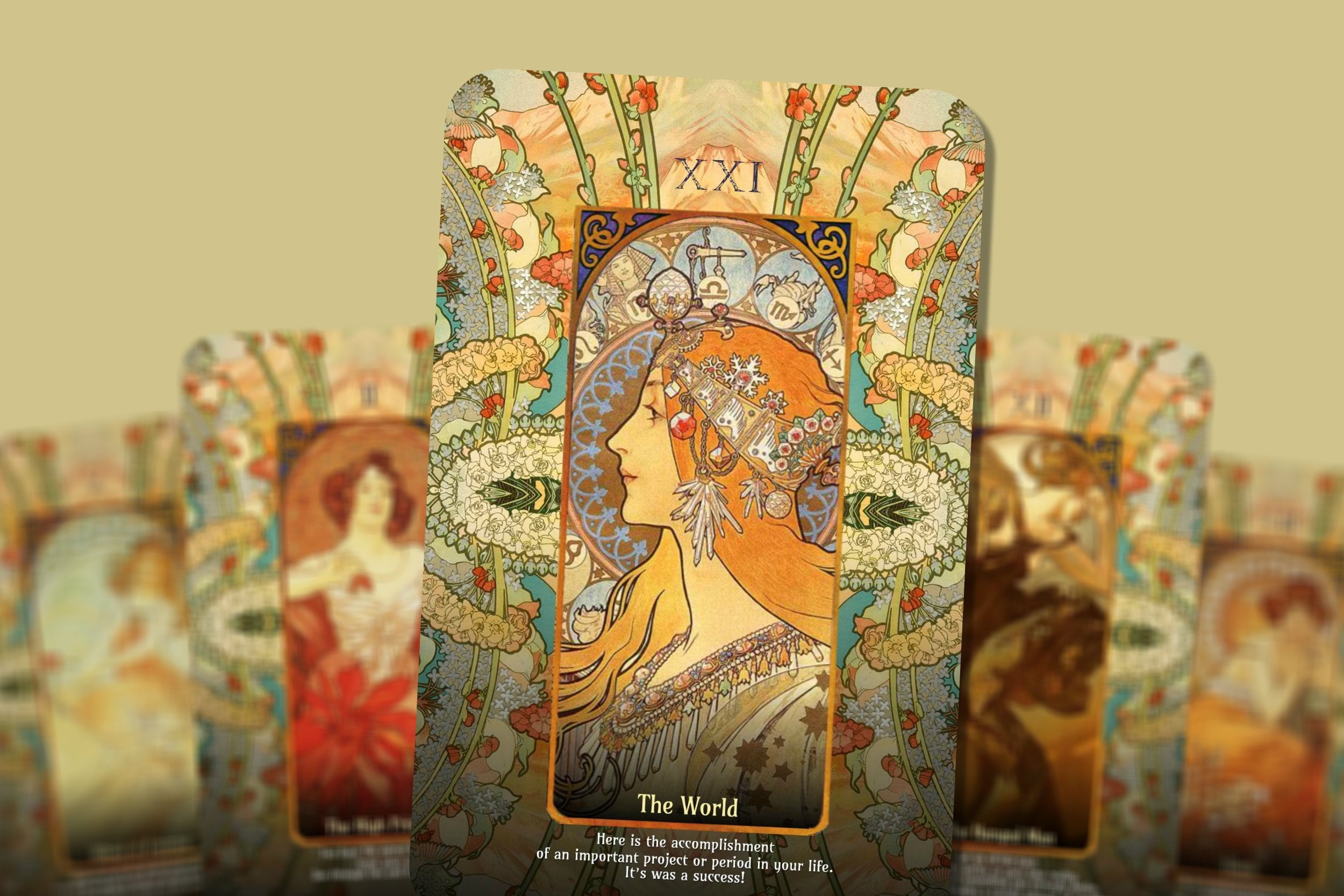The image is a photograph of five decorative tarot cards set against a yellow background. The central card is prominently featured, with the remaining four cards partially blurred in the background. This central card has a vibrant, intricate border adorned with vines, small red flowers, and other ornate designs in greens, beige, and peach. At the top of this card, "XXI" is displayed, signifying the card known as "The World." In its center, a stylized drawing depicts a woman in profile. She has orange hair and wears a head wrap adorned with feathers, jewelry, and gems. Her pale face is highlighted with a scarf on her head. Beneath her image, in white letters, it says, "The World," followed by the message, "Here is the accomplishment of an important project or period in your life. It was a success." The overall artwork of the cards is unique and detailed, suggesting they are special tarot cards with significant decorative appeal.